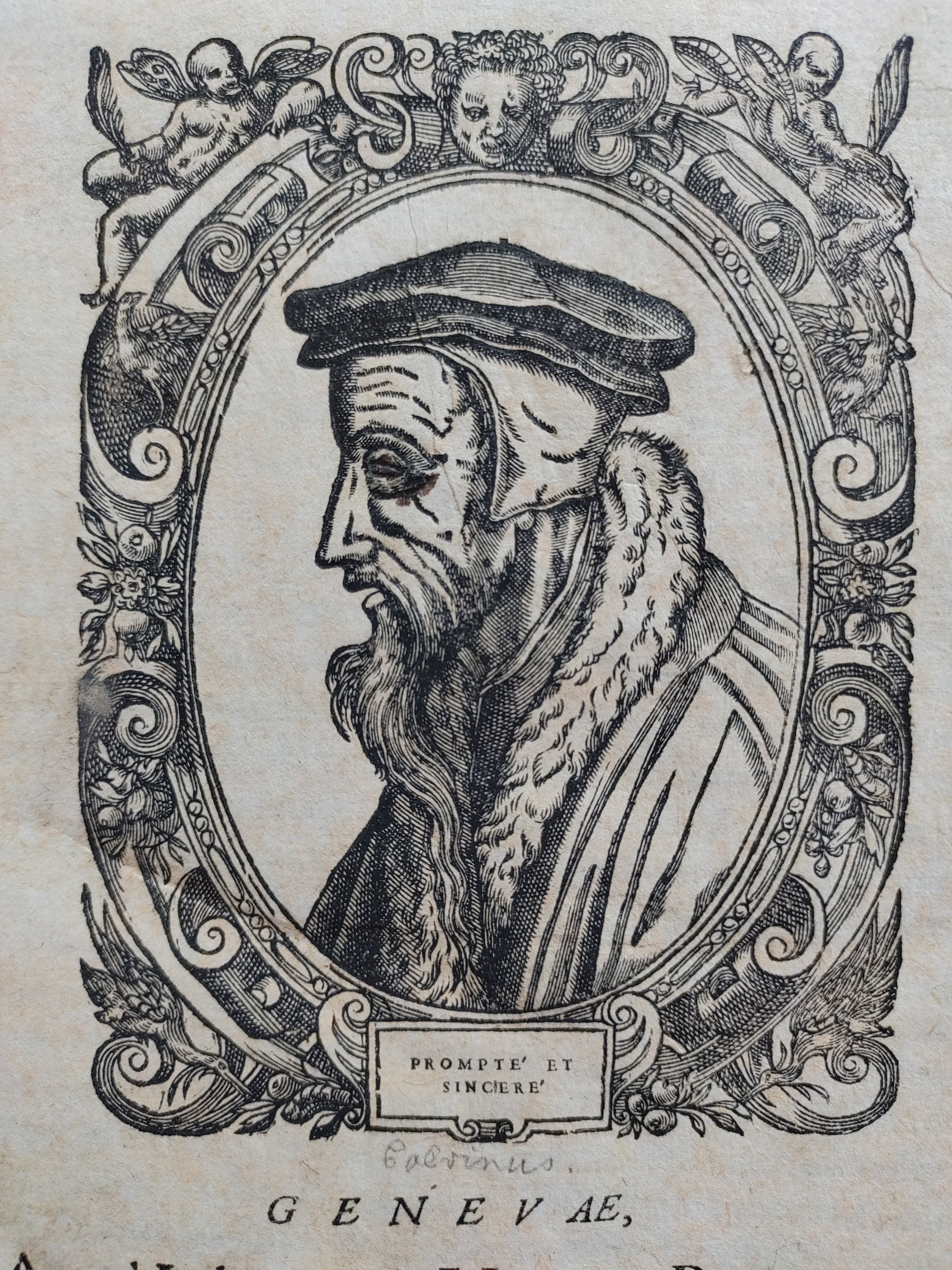The image depicts an intricately detailed etching of an elderly man, showcasing a profile view from his left side. This portrait is framed within an ornate oval border adorned with cherubs, scroll-like lines, and fruit motifs, indicative of classical design elements. The man, whose solemn profile is highlighted by prominent facial wrinkles, wears a dark, possibly French-style cap and a fur-collared coat. His long, flowing beard stretches down to his chest, adding to his distinguished appearance. The entire etching is rendered in black ink against a cream background, creating a stark contrast that emphasizes the intricate details. Beneath the man's portrait, the inscriptions include "C-A-L-V-I-N-U-S" in handwritten text, followed by "Prompt prompte et sincere" and "G-E-N-E-V-A-E," suggesting a historical or literary significance to the piece.